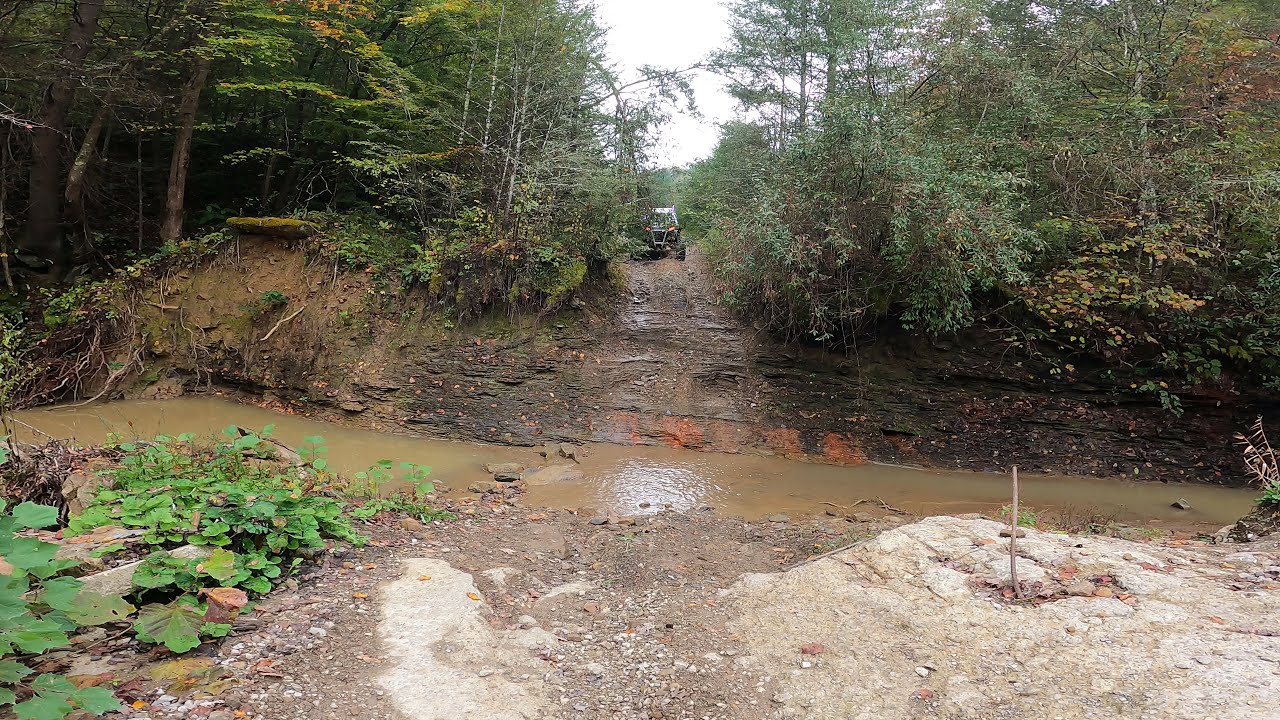This image captures a serene, off-road scene in a wooded area. The bottom quarter of the image features a tan shoreline with some greenery on the left. Running horizontally about a third of the way up the image is a small, brown creek, whose banks are lined with exposed roots and rocky, dirt embankments. Tall trees with green, yellow, and orange leaves flank both sides of the scene, their roots trailing down the slopes to the water. Centered near the top of the image, a dirt path cuts through the vegetation, descending towards the creek. An off-road utility vehicle, possibly an ATV or tractor, makes its way down this path, its red lights visible. The overall impression is one of a damp, potentially post-rainfall setting, with an overcast sky contributing to the earthy tones and lush greenery typical of a forest or tropical rainforest environment.